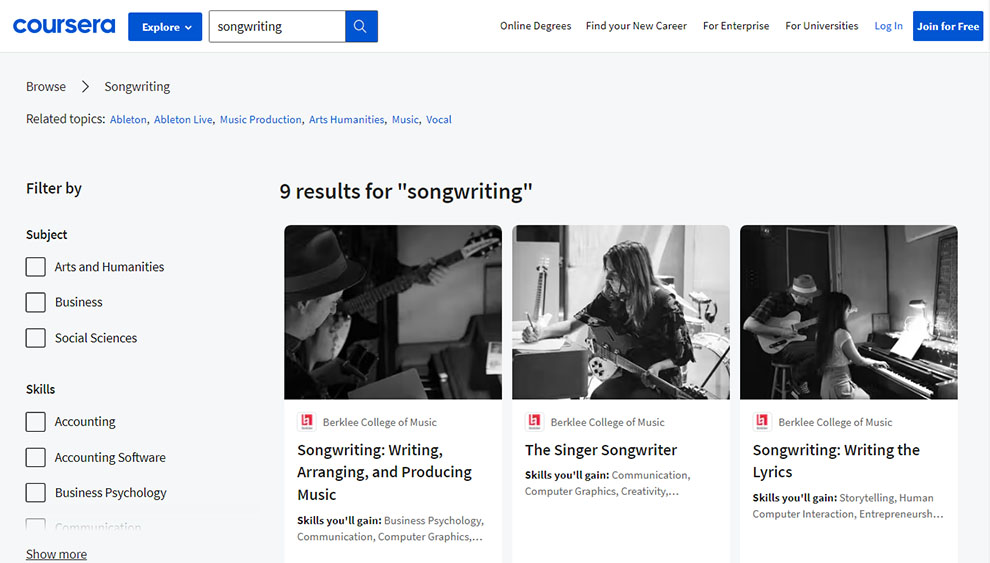This screenshot captures the homepage of Coursera, a popular online learning platform, displayed on a widescreen desktop or laptop computer. The interface showcases options for exploring various courses designed to help users learn new skills or enhance their existing knowledge. 

In the upper left corner, the Coursera logo is prominently displayed next to an "Explore" button. Adjacent to the logo is a search bar where a user is actively searching for "songwriting". To the far right of the search bar lie several buttons leading to specific sections: "Online Degrees," "Find Your New Career," "For Enterprise," "For Universities," "Log In," and "Join for Free."

Below the primary navigation bar, the page further breaks down into sections that allow users to browse topics related to "Songwriting," such as "Ableton," "Ableton Live," "Music Production," "Arts," "Humanities," "Music," and "Vocal."

The screenshot lists nine results for "songwriting" courses. Noteworthy among them are multiple offerings from the Berklee College of Music, including:
1. "Songwriting: Writing, Arranging, and Producing Music," where participants can gain skills in business psychology, communication, and computer graphics.
2. "The Singer-Songwriter" course which aims to enhance skills in communication, computer graphics, creativity, and songwriting.
3. "Songwriting: Writing the Lyrics," designed to develop skills in storytelling, human-computer interaction, and entrepreneurship.

On the left side of the screen, filter options are shown to narrow down course selections by subjects such as "Arts and Humanities," "Business," "Social Sciences," "Accounting," "Accounting Software," and "Business Psychology."

The page features a clean, minimalist design with a white background and contrasting black text, ensuring readability and ease of navigation.